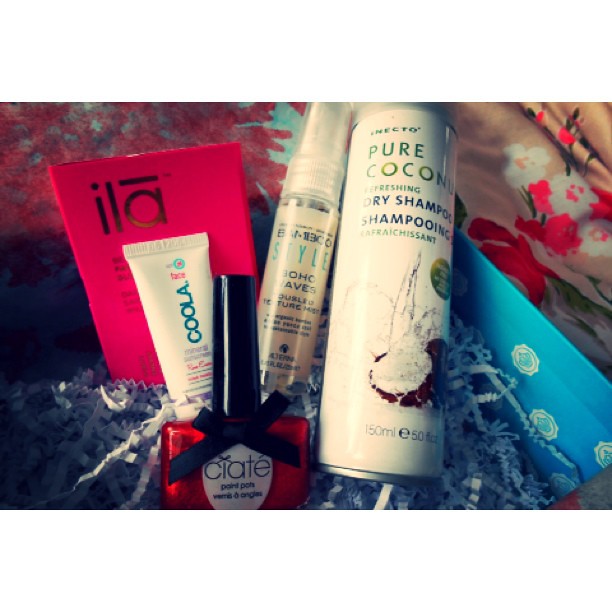The image features a high-quality, thick blue cardboard gift box with a white emblem on the lid, which is open to reveal a floral patterned interior. Inside, a layer of shredded, crinkled paper nestles five distinct beauty and self-care products. At the forefront is a red glass nail polish bottle with a black lid, branded "Ciaté." Behind it sits a white tube labeled "Kula." Parallel to Kula is a small pink rectangular box marked "Isla." A clear pump spray bottle labeled "Style" is positioned in the center, although glare obscures some details. Completing the collection is a white aerosol can of "Pure Coconut Dry Shampoo" featuring a depiction of a coconut with water splashing from it. The overall setup rests on a decorative fabric adorned with pink, red, and white flowers.